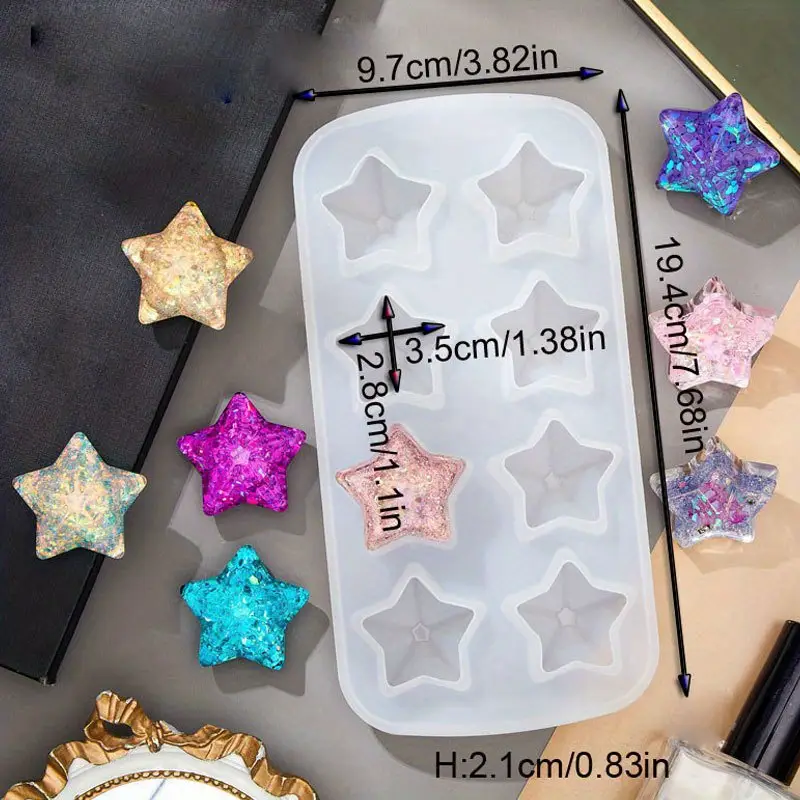The image features a white or clear tray designed to create star-shaped items, likely used for crafting or baking. The tray includes detailed measurements along its sides, labeled in both centimeters and inches: 9.7 cm (0.82 inches) and 19.4 cm (7.68 inches). The height is indicated as 2.1 cm (0.83 inches). The tray has cutouts for the stars, and the picture showcases a variety of colorful star-shaped samples, possibly made using the tray. These stars come in vibrant hues including pink, blue, tan, purple, magenta, turquoise, dark purple, chartreuse, silver, and gold. The stars are visually striking, with some appearing sequined or glittery, suggesting the possibility of incorporating such materials into the molding process. The tray holds eight star shapes at a time, and the overall scene is set on what appears to be a crafting table, indicating this tool's versatility for various creative projects.